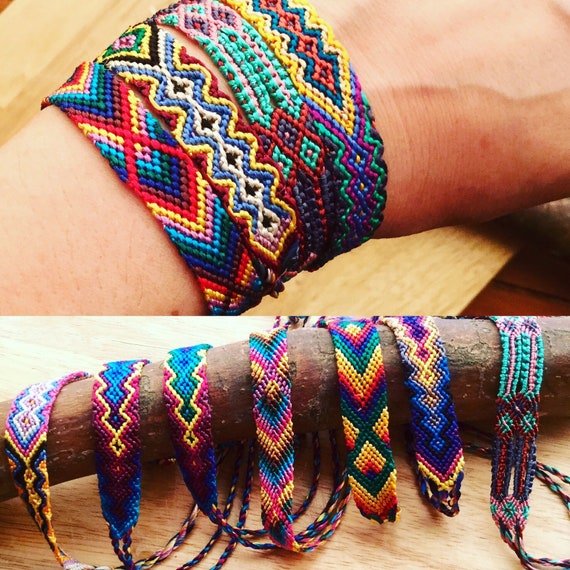The image is a composite of two photographs, meticulously stitched together. The top photograph showcases a close-up of a person's wrist, adorned with a series of thin, colorful, hand-woven friendship bracelets. These bracelets display intricate patterns such as diamonds, zigzags, and other unique designs, weaving a tapestry of multicolored threads. The wrist rests on a wooden surface, likely a table. Below, the second photograph presents these handmade bracelets untied and neatly arranged side-by-side along a long piece of wood, resembling a tree branch, which is also placed on a wooden table similar to the one above. The juxtaposition highlights the versatile beauty of the bracelets; their tactile charm and detailed craftsmanship are evident in both their stacked form on the wrist and their spread-out arrangement on the branch.